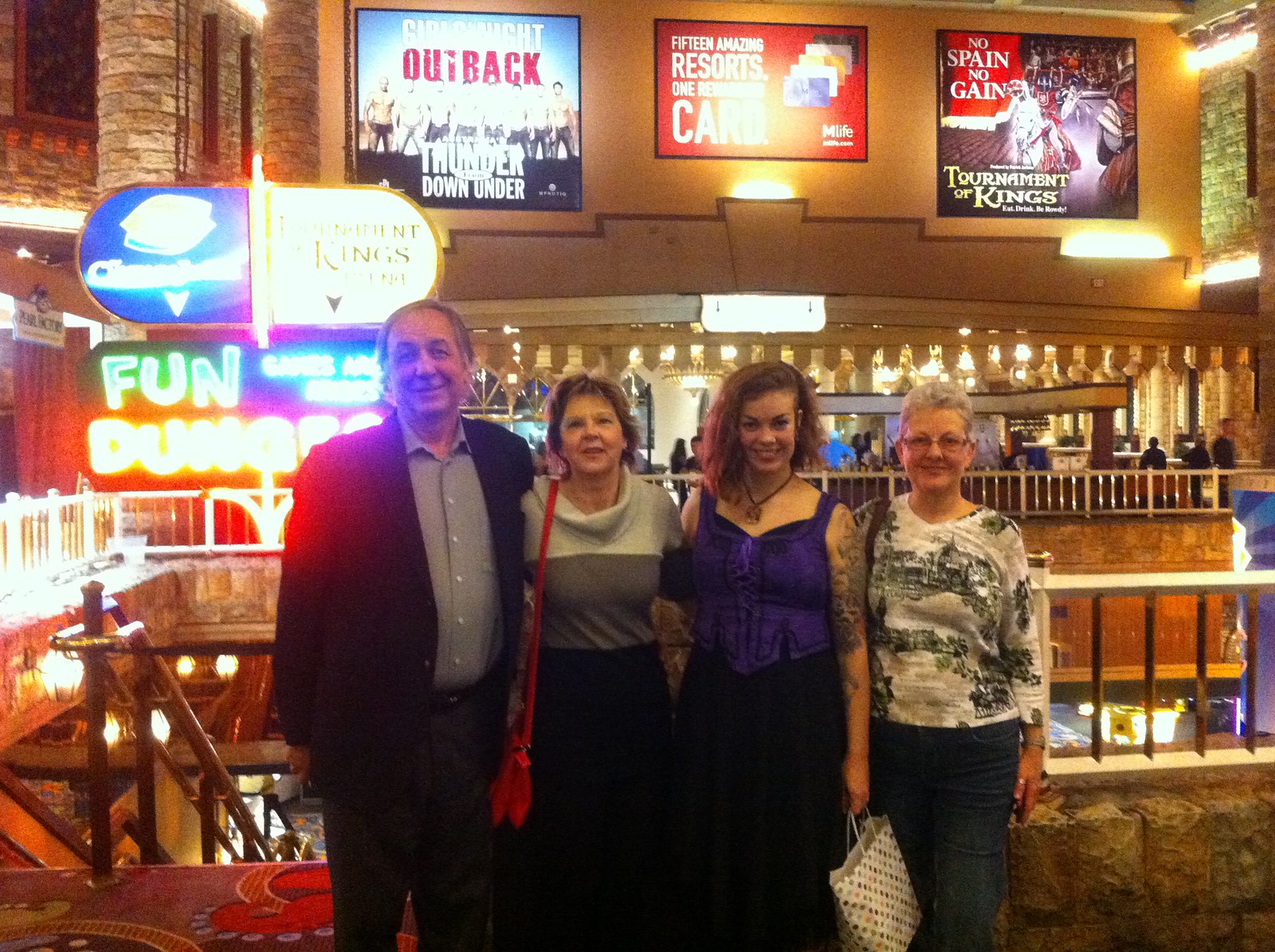In this vibrant and lively image set in a dimly lit restaurant or event venue, four individuals stand together in front of a yellowish-brick wall adorned with neon lights and various posters. The atmosphere is warm with a distinctly yellow hue emanating from the interior lighting and complemented by numerous neon signs in the background that amplify the spirited ambiance. To the left, a man in a blue sports coat paired with gray pants smiles warmly. Beside him, a woman with short hair dressed in a gray sweater and holding a red purse embraces another woman sporting a blue tank top, tattoos, a black skirt, and curly brown hair. This woman, with a cheerful expression, also has a distinctive polka-dotted bag with hints of purple, green, and yellow. Next to her stands an older lady with short gray hair, wearing a white and black top and blue jeans, accessorized with glasses and a silver wristwatch. Behind these individuals, the wall is decorated with diverse signage, including a notable "FUN" sign in yellow and blue, and various posters such as "Outback Thunder Down Under" in red and white text, contributing to an engaging backdrop filled with colors and energetic details. The floor beneath them carries a mix of red and yellow tones, enhancing the scene's eclectic and festive vibe.